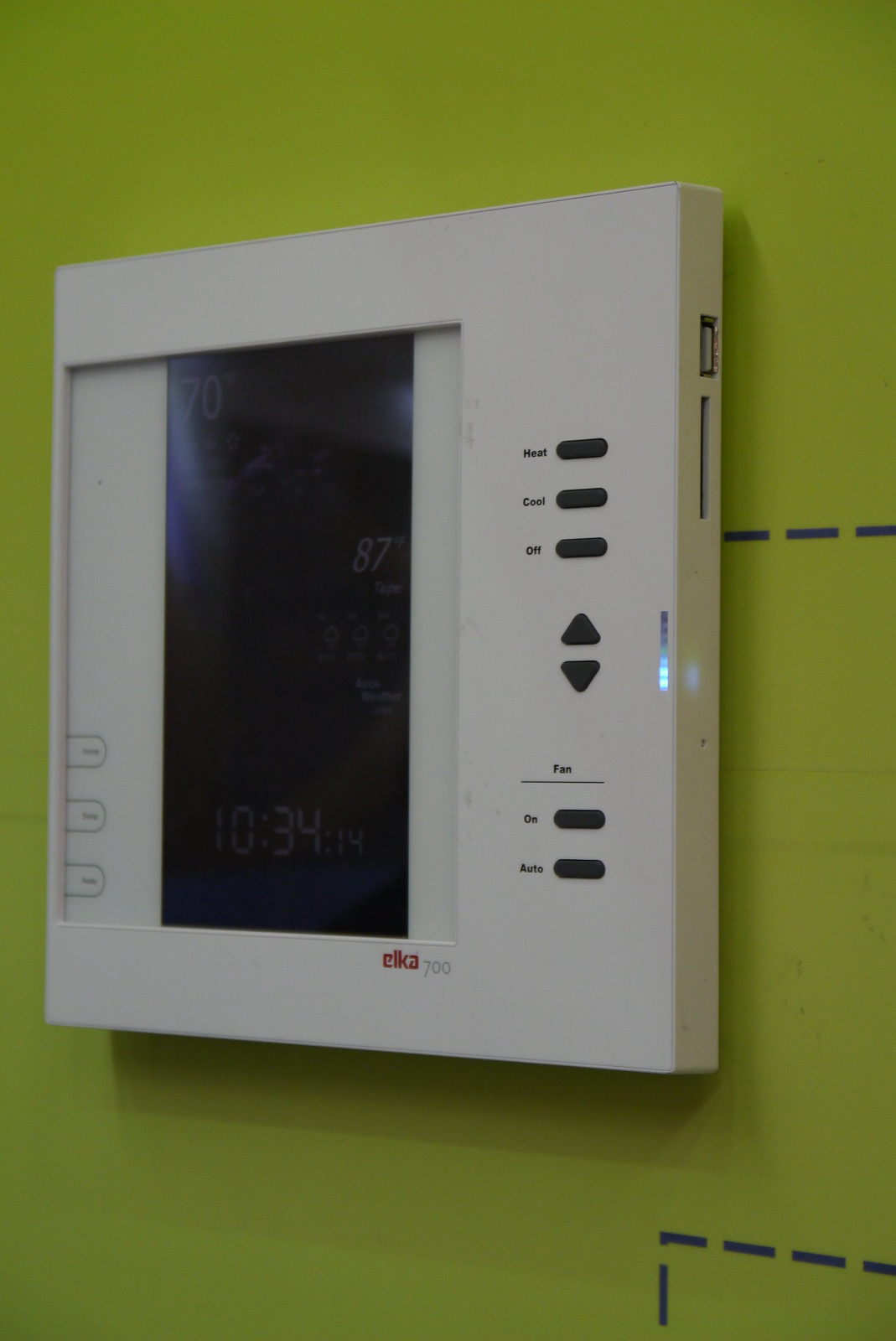The image displays an electronic control panel set against a white or green background. Prominently featured is the text "Elka 70" in red, indicating the device model. The control panel has a black background with various functions and settings. There is a fan mode option which can be toggled between "On" and "Auto." The interface includes up and down arrows for adjusting settings, along with separate buttons for heat, cool, and off functions. On the left side of the panel, there are three additional buttons whose labels are not legible. The screen also displays the current time as "10:34:14."